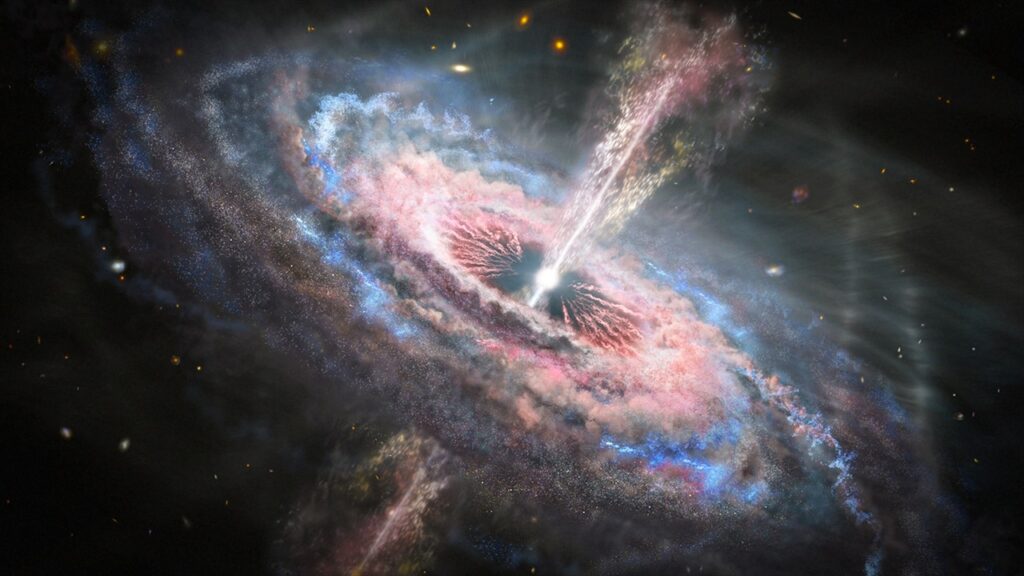The image presents an artistic rendering of a cosmic event within a spiral galaxy. The galaxy features a vibrant explosion of colors, where the edges transition from blue to vivid hues of red and yellow towards the center. At the very core lies a luminous ball of light emitting radiant red and yellow beams both upward and downward, accentuated by small flecks of gold. Surrounding the central light, to its left and right, are red tendrils that stretch towards, yet don't quite meet the central glow. The scene is set against a deeply black background, reminiscent of the vastness of space, with dust clouds in shades of gray, pink, and blue fanning out from the center. Speckled lights resembling stars add to the celestial ambiance. The swirling vortex at the core, with its interplay of pink, blue, red, and orange hues, encapsulates a vivid sense of motion and mystique, further emphasized by beams of pink and white light piercing through from top to bottom, creating an impression of dynamic, otherworldly energy.